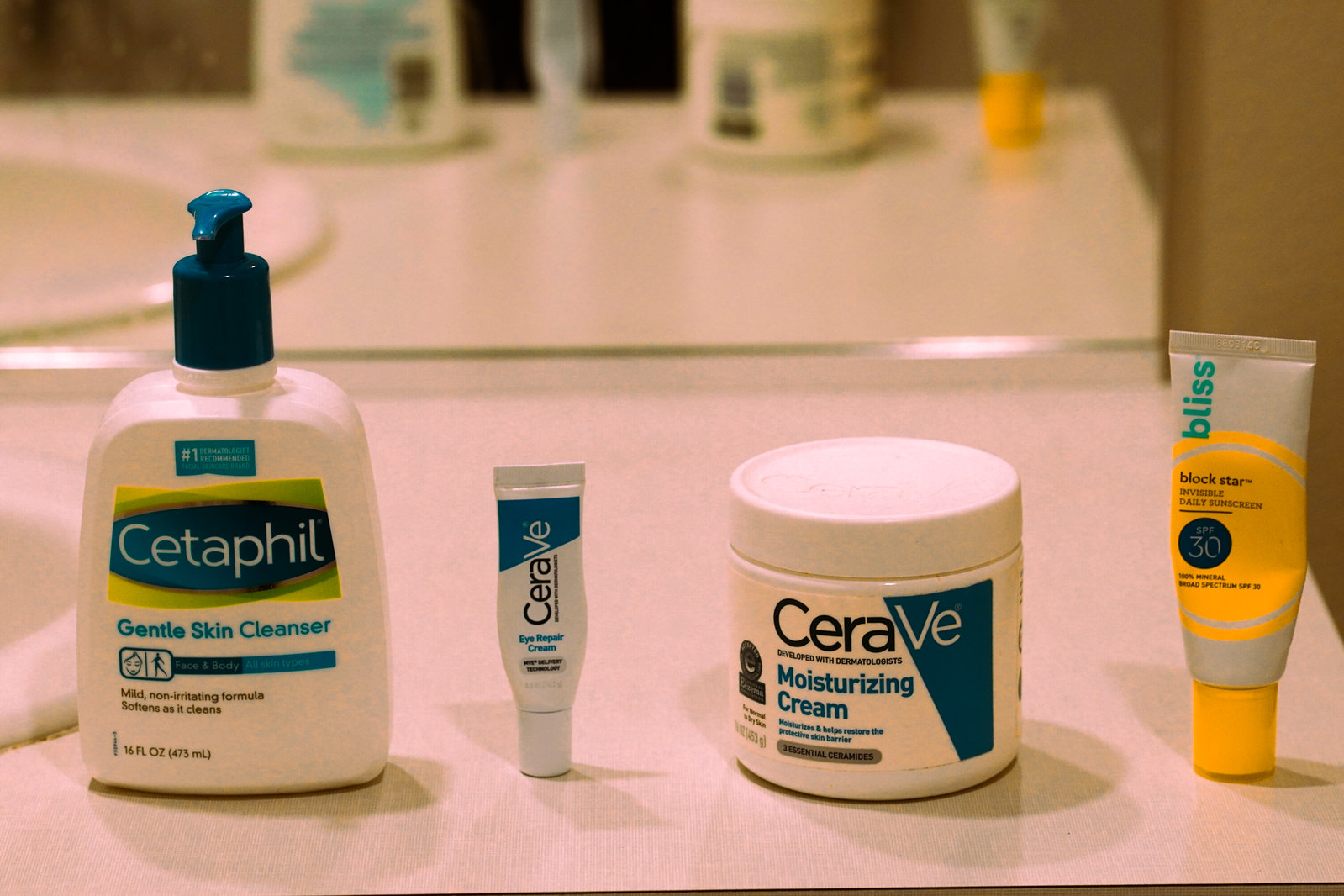On a plain white laminate bathroom countertop, various skincare products are neatly arranged beside a white ceramic sink basin. The rectangular silver mirror above reflects the collection of items, emphasizing the counter’s practical, no-frills design. 

To the far left stands a 16-ounce (473ml) Cetaphil Gentle Skin Cleanser bottle, distinguished by its white body and blue cap. The label promises a mild, non-irritating formula suitable for softening as it cleans.

Next to it is a small, tube-shaped container resembling a ChapStick, but it is actually CeraVe Eye Repair Cream. The tube features dark blue and white elements with black print in a grey oblong bubble, indicating its specialized purpose for eye care.

Adjacent is a short, wide jar-like bottle from CeraVe, labeled as Moisturizing Cream. The packaging highlights its dermatologist-developed formula, designed to moisturize and help restore the skin’s protective barrier with three essential ceramides. The exact volume of the cream remains indistinct.

On the far right of the arrangement is a slightly larger tube from the brand Bliss. Marked with a stylized yellow sun and the phrase "Block Star," this product is an Invisible Daily Sunscreen with SPF 30. The packaging, featuring lowercase green font and black print, emphasizes its 100% mineral, broad-spectrum protection.

This orderly display of skincare products showcases a curated selection aimed at maintaining and protecting skin health.